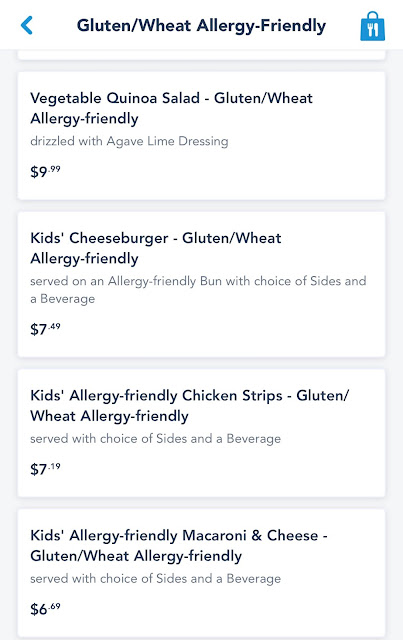Here is the cleaned-up and descriptive caption for the image:

---

The image depicts a results page with a vertical, rectangular layout. The background is a very pale blue or pale gray, featuring a series of horizontal white boxes arranged vertically. Each box contains a menu item, complete with its price and description. 

At the top of the page, in bold black text, it reads "Gluten/Wheat Allergy Friendly." Next to this text, there's a small blue tote bag icon with a white knife and fork inside.

1. **Vegetable Quinoa Salad - Gluten/Wheat Allergy Friendly**  
   Description: Drizzled with agave lime dressing.  
   Price: $9.99

2. **Kids Cheeseburger - Gluten/Wheat Allergy Friendly**  
   Description: Served on an allergy-friendly bun with a choice of sides and a beverage.  
   Price: $7.49

3. **Kids Allergy-Friendly Chicken Strips - Gluten/Wheat Allergy Friendly**  
   Description: Served with a choice of sides and a beverage.  
   Price: $7.19

4. **Kids Allergy-Friendly Macaroni and Cheese - Gluten/Wheat Allergy Friendly**  
   Description: Served with a choice of sides and a beverage.  
   Price: $6.69

---

This detailed caption provides a thorough description of the content and layout of the menu page while maintaining clarity and structure.